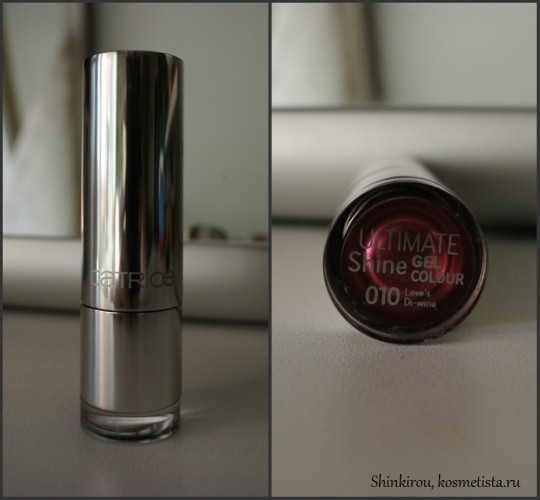The image is divided into two vertical sections, each depicting a silver tube of lipstick from different angles against a blurred gray background. On the left side, the lipstick stands upright, showcasing a sleek, closed container with the brand name "Patrice" faintly visible in gray font. The design features a larger top section and a dividing line where the tube would open. On the right side, the lipstick tube is lying on its side, revealing the bottom part of the container, which is labeled "Ultimate Shine Gel Color 010" in a mix of uppercase and lowercase letters. Below this, in a smaller, difficult-to-read font, it says "Loves DI-Wine," along with the text "ShinkiroCosmetista.ru" at the bottom. The overall background remains consistent, enhancing the focus on the detailed product features.